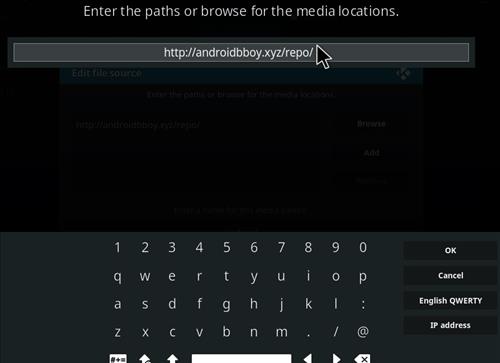The image appears to be a screen capture featuring a user interface with a predominantly black and gray background. At the top of the image, there is gray text that reads, "Enter the paths or browse for the media locations." Below this, there is a gray input box displaying a web address, "androidboy.xyz/repo," accompanied by a visible black mouse cursor.

Faintly visible in the background, behind this central section, is a teal box containing the text "Enter file source," along with additional white font that is partially obscured.

Towards the bottom of the image, there is a large dark gray square filled with numerous white characters. This section appears to be a virtual keyboard, featuring a number pad with digits from 0 to 9, alphabetical letters, and various symbols. At the lower part of this keyboard, there are navigation keys, including back arrows, forward arrows, an 'x' button, and an up arrow.

Adjacent to this gray square are four black boxes with slightly pixelated white text. The labels on these boxes read as follows:
1. "OK"
2. "Cancel"
3. "English QWERTY"
4. "IP Address"

It should be noted that in the text "IP Address," only "IP" is capitalized.

The background image is blurred and overlaid with other UI elements, making it indistinct and unremarkable. There are no additional significant details to note in this image.